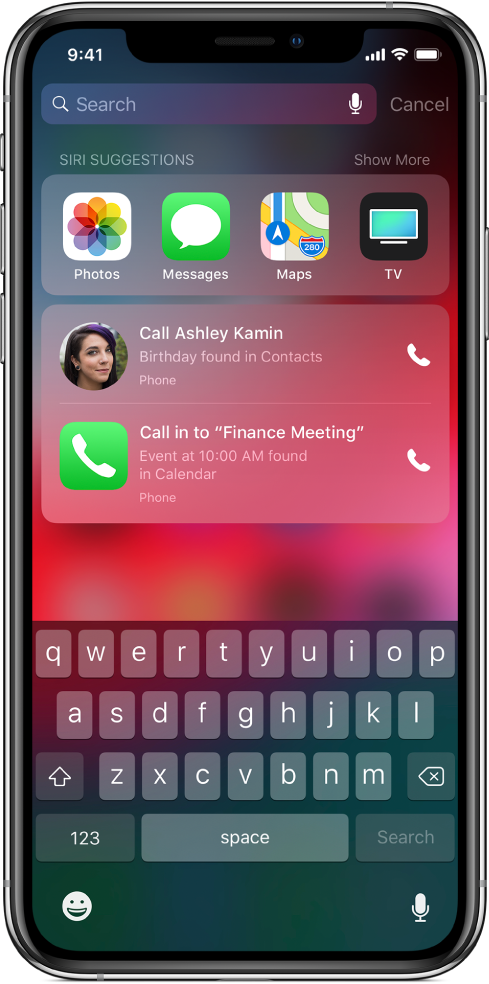The image displays a cell phone screen with the notification and information drop-down menu revealed. 

**Screen Details:**
- **Top Left Corner:** The time is shown as 9:41.
- **Top Right Corner:** Displayed are four white signal bars, a white Wi-Fi icon, and a fully charged white battery icon.

**Main Section:**
- At the top center, there is a search bar containing a magnifying glass icon and the text "Search". To the right of this bar is a microphone icon and a "Cancel" button.
- Below the search bar, the text "Siri Suggestions" is prominently displayed in white.
- Following this, several semi-transparent icons are listed vertically:
  1. **Photos:** A white box with a multicolored flower icon, labeled "Photos".
  2. **iMessages:** A green box featuring a white chat bubble, labeled "iMessages".
  3. **Maps:** An icon representing a map.
  4. **TV:** A black icon with a blue television symbol.
- A separate text box shows an image of a woman with dark brown hair, labeled "Ashley Kamin" (K-A-M-I-N) with the note "Birthday found in contacts and phone" and an adjacent phone receiver icon on the right.

**Further Details:**
- Another text box below contains information about a call scheduled: "Call into finance meeting, event at 10 a.m., found in calendar," with a phone icon to the right.
- At the bottom, a QWERTY keyboard is visible with the standard layout:
  - **Top Row:** Q-W-E-R-T-Y-U-I-O-P
  - **Second Row:** A-S-D-F-G-H-J-K-L
  - **Third Row:** Z-X-C-V-B-N-M with a backspace arrow next to 'M' and a shift arrow next to 'Z'
  - Below these rows are buttons for "1-2-3," a space bar, "Search," an emoji icon, and a microphone icon. The keyboard background is black.

**Background and Design:** 
- The background of the icon and text boxes is blurred, displaying a mix of reddish pink and blue-black colors.
- Near the top of the screen, to the right of "Siri Suggestions," there is a "Show More" option.

This detailed description captures the content and layout of the cell phone screen as depicted in the image.